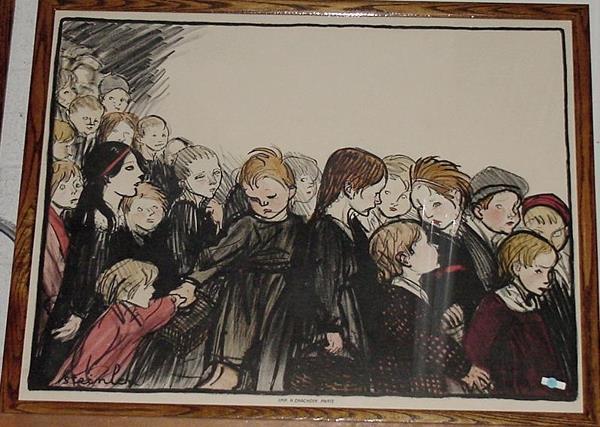This painting depicts a somber scene of approximately 30 school-aged children, seemingly around 10 to 12 years old, standing in a line or moving in a procession from left to right. Most of the children are dressed in muted, dark colors, predominantly black. Notably, one girl at the bottom right wears a dark red sweater, and another child sports a long-sleeved red shirt, adding minimal pops of color to the otherwise somber palette. One young girl in a lighter pink dress stands out, reaching out to hold the hand of another child. The children's expressions are uniformly solemn or frightened, contributing to a sense of melancholy or fear. While the background is bare and indistinct, the children's attire and appearance suggest an older historical era. Their hair ranges from light blondes and reds to a few with darker hues, and many of the girls have their hair up, while some boys wear hats. The minimalistic detail in their facial features, marked only by simple lines and circles, heightens the overall somber and eerie atmosphere, conjuring the feeling of a grave or funeral-like procession.